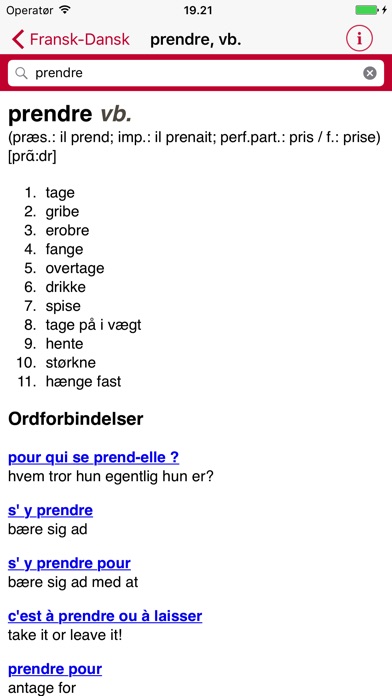This image is a screenshot from an iPhone, evidenced by the recognized battery icon in the top right corner and the Wi-Fi symbol in the top left. It reveals a dictionary or translation page in French, with someone looking up the verb "prendre." The header of the page reads "Fransk-Dansk" followed by "Prendre," indicating a French-Danish translation. The page is structured with black text primarily for definitions and blue text for links. At the top left, the word "Operator" is displayed next to the Wi-Fi symbol, and the time is shown as 19:21. The result includes different verb tenses of "prendre," followed by a numbered list of associated words. The page layout is neat, with a light blue background, and features additional elements like a red circular information icon and a red-lined search bar. Links at the bottom prompt further exploration of related terms.